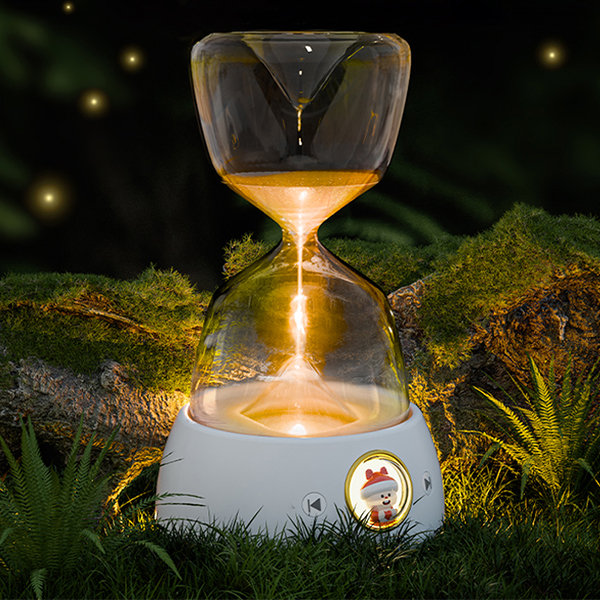The image depicts an hourglass-shaped object exuding a warm, golden glow, with a distinct yellow, orange, and amber hue. Unlike a traditional hourglass filled with sand, this one appears to have glowing elements inside. The top of the glass structure is white, seamlessly blending into the smooth white plastic base. A thick white band encircles the base, featuring a small circular emblem with a charming cartoon character, resembling a Christmas elf or a mini Santa Claus, dressed in a red and white outfit. Adjacent to the character are back and forward buttons on either side of the circle. This entire scene is situated outdoors, with the hourglass set on a mossy, grassy patch, surrounded by ferns and other greenery. The background is a dark night sky, illuminated by what looks like fireflies or stars, adding to the enchanting atmosphere. The glowing hourglass light bathes the surrounding vegetation in a gentle, warm glow, enhancing the overall magical and serene ambiance of the scene.